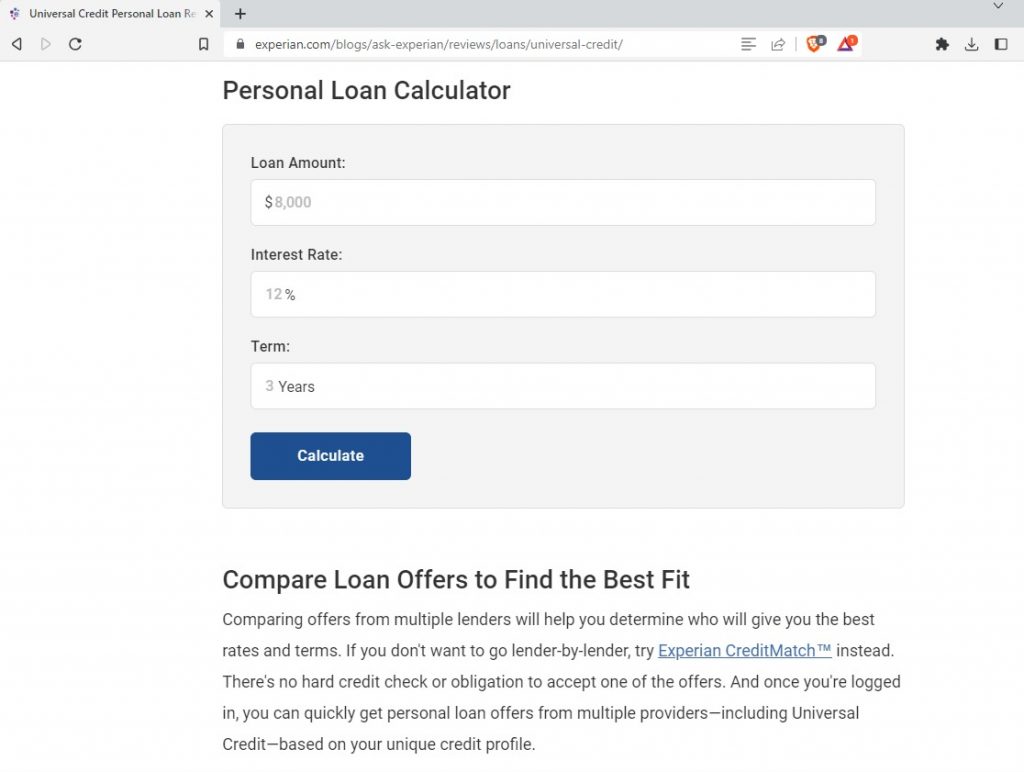The webpage screenshot from Experian displays their personal loan calculator. The URL in the page header reads: "Experian.com/blogs/ask-experian/review/loans/universal-credit/calculator." On the page, there's a section titled "Personal Loan Calculator" featuring an input field where a loan amount of $8,000 is entered, an interest rate field showing 12%, and a term field indicating 3 years. Below these inputs, a blue "Calculate" button awaits a click to compute the loan details based on the provided information.

Additionally, the page includes an informational section encouraging users to compare loan offers to find the best fit. This section highlights the benefits of comparing loan offers from multiple lenders to secure the best rates and terms. It mentions the use of Experian Credit Match, a tool that lets users compare offers without triggering a hard credit check. The description underlines the simplicity of obtaining personal loan offers from various providers, such as Universal Credit, tailored to the user's credit profile. Overall, this webpage serves as a tool for calculating personal loan repayments and promotes the comparison of different loan offers to achieve the most favorable deal.